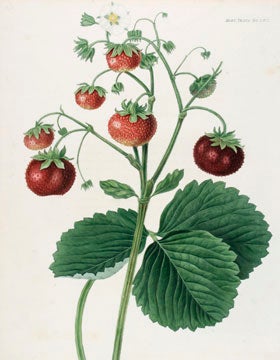The illustration, resembling a vertically aligned card measuring approximately 2 inches wide by 3 inches tall, depicts a strawberry plant on an off-white or pale gray background with a pinkish hue. Emerging from the bottom center, a single thick green stem rises to the midpoint, where it branches out into three large leaves on the right and one on the left, with two smaller, rounded leaves above them. These leaves are a vibrant green, lending a lifelike quality to the plant. The stem further divides into smaller branches, each supporting bulbous, textured strawberries in various stages of ripeness—from lighter, less mature berries at the top to deeper red, fully ripe ones towards the bottom. A single white flower crowns the top of the plant, symbolizing the beginning of the fruiting process. Faded fine print in the upper right corner of the card adds a touch of authentic, vintage charm, though its content is unreadable.